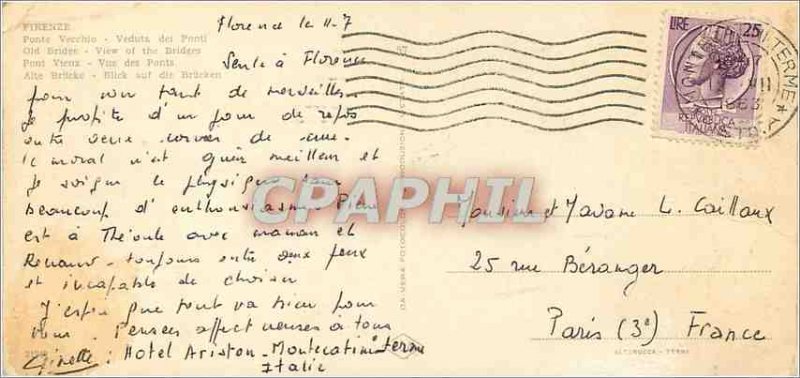The image depicts an aged, ivory-colored postcard with visible stains. The postcard features handwritten text in black ink on the left side, written in cursive and difficult to read, likely French. On the right side, at the top, there is a postage stamp with a purple background, depicting a woman's left-facing profile wearing a crown. Next to the stamp are squiggly lines indicating it has been mailed. The handwritten address on the bottom right reads "25 rue Berger, Paris, France." The postcard also shows signs of aging, particularly yellowing around its edges. A semi-transparent watermark in the middle reads "CPAPHIL," with slightly glowy edges that stand out against the aged background.